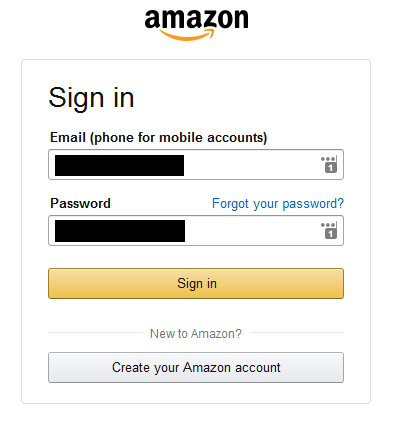This image depicts the Amazon sign-in page. The layout includes a prominent black rectangle at the center with fields for "Email or mobile phone number" and "Password". To the right, there's an ellipsis icon (three dots) followed by a number "1". Below the password field, there's a blue link labeled "Forgot your password?". Another black rectangle follows, and at the bottom of the page, a yellow rectangle button labeled "Sign-In". Beneath that, text reads "New to Amazon?" and there's another rectangle stating "Create your Amazon account". The edges of the image are lined with various design elements to frame the form, and overall, the page facilitates user login and account creation for Amazon.